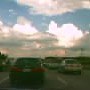In the late afternoon, between 5 p.m. and 6:30 p.m., a serene scene unfolds on a bustling highway. Four cars advance steadily towards the horizon, where a faint, setting sun casts a soft glow, suggesting a tranquil end to the day. The sky above transitions into a gentle bluish hue, peppered with numerous clouds, adding depth and texture to the twilight. Beyond the vehicles, possibly obscured by their presence, lies the hint of a distant mountain at the horizon's edge. The scene exudes a sense of calm and order, with all traffic moving in unison towards a single direction, unmarred by any counter flow. The composition captures the essence of an early evening journey, where the day's end meets the promise of night.